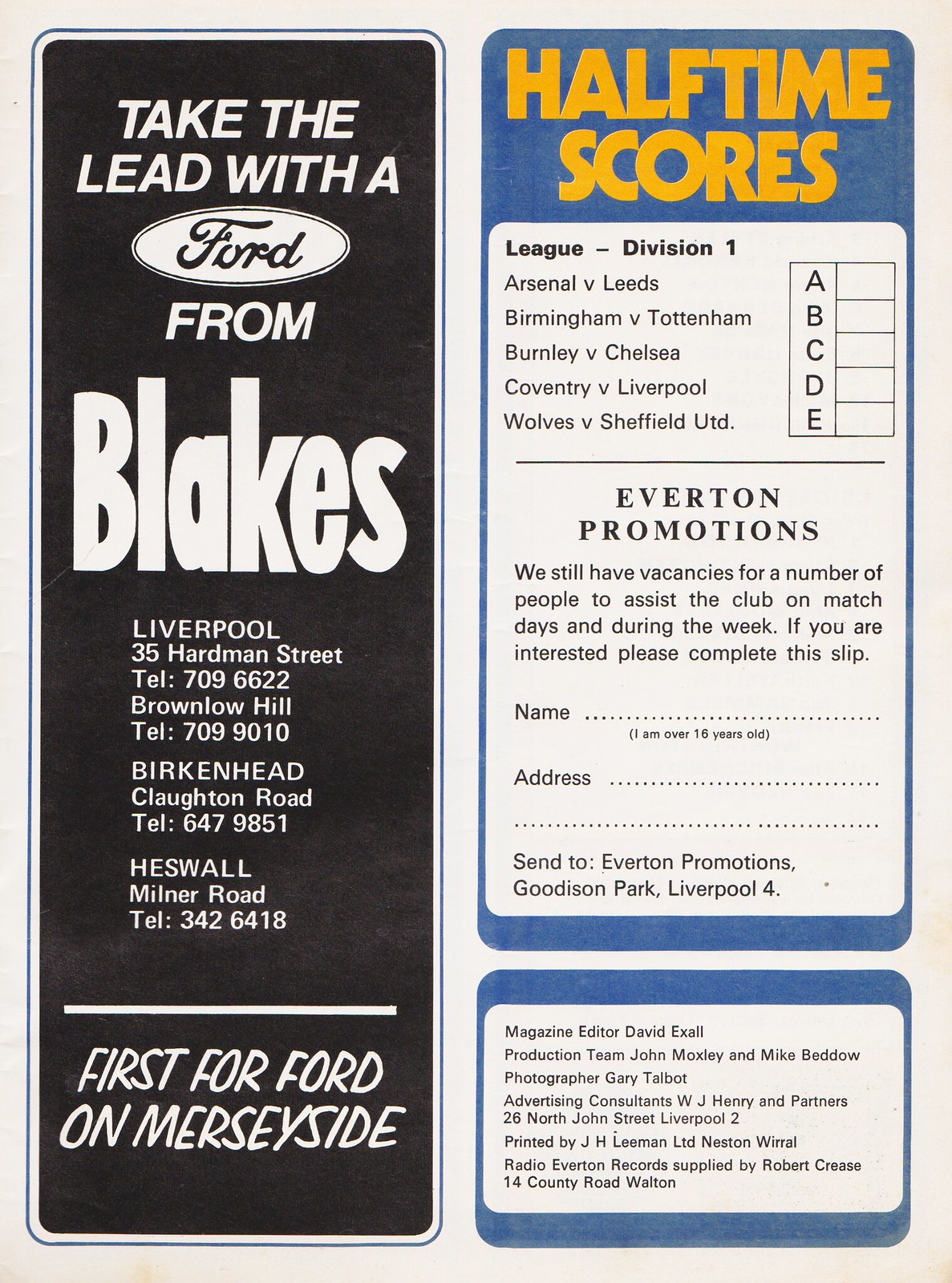This is an advertisement scan from an old magazine, divided into two distinct sections, each featuring prominent content. The left half, set against a black background, prominently displays a car dealership ad with the headline "Take the Lead with a Ford from Blake's." Blake's, a Ford dealership, lists multiple locations: Liverpool at 35 Hardman Street, Brownlow Hill, Burkhead on Clayton Road, and Heswell on Milner Road. Contact numbers are provided for each location. Below these details, a bold tagline declares "First for Ford on Merseyside."

On the right half of the page, the content shifts to football (soccer) with a scorecard-like section. At the top, in yellow text, it reads "Half-Time Scores," followed by match details in black text within white boxes. The listed League Division 1 matches are Arsenal vs. Leeds, Birmingham vs. Tottenham, Burnley vs. Chelsea, Coventry vs. Liverpool, and Wolves vs. Sheffield United. Beneath this, a line of promotions invites readers to assist the club on matchdays and during the week, instructing interested individuals to complete the provided form. The bottom section includes publication details, such as the magazine editor and printing information.